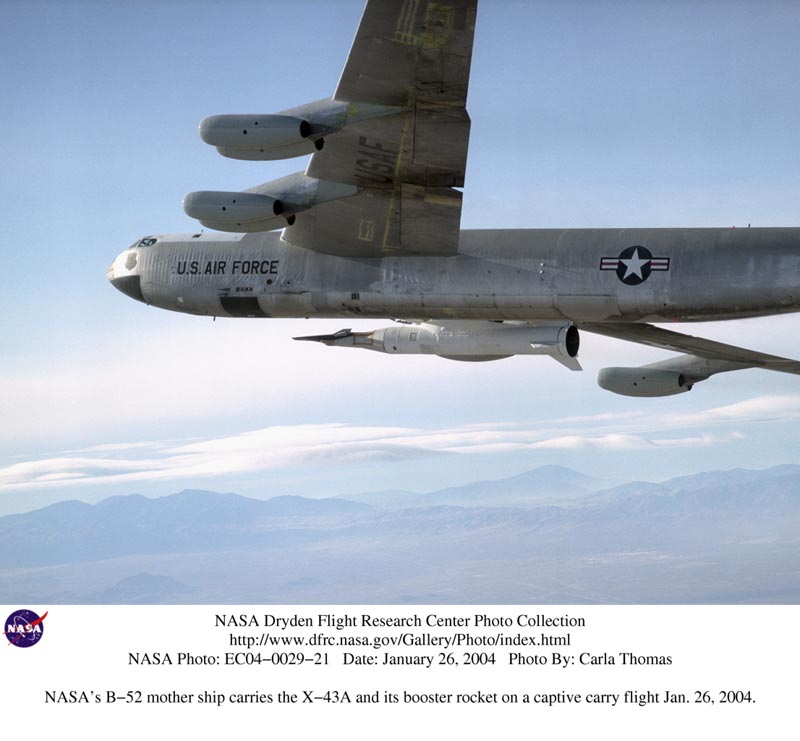The photograph captures a striking scene of a U.S. Air Force jet, specifically NASA's B-52 mothership, flying above the clouds with a large missile, the X-43A and its booster rocket, secured underneath. The vast expanse below, partially obscured by a haze of clouds, reveals distant mountain ranges, adding grandeur to the image. Text at the bottom of the photo provides essential details: "NASA Dryden Flight Research Center Photo Collection, http://www.dfrc.nasa.gov/gallery/photo/index.html, NASA photo EC04-0029-21, date January 26, 2004, photo by Carla Thomas." This image, taken on January 26, 2004, expertly photographed by Carla Thomas, showcases a significant moment in aerospace research and technology.